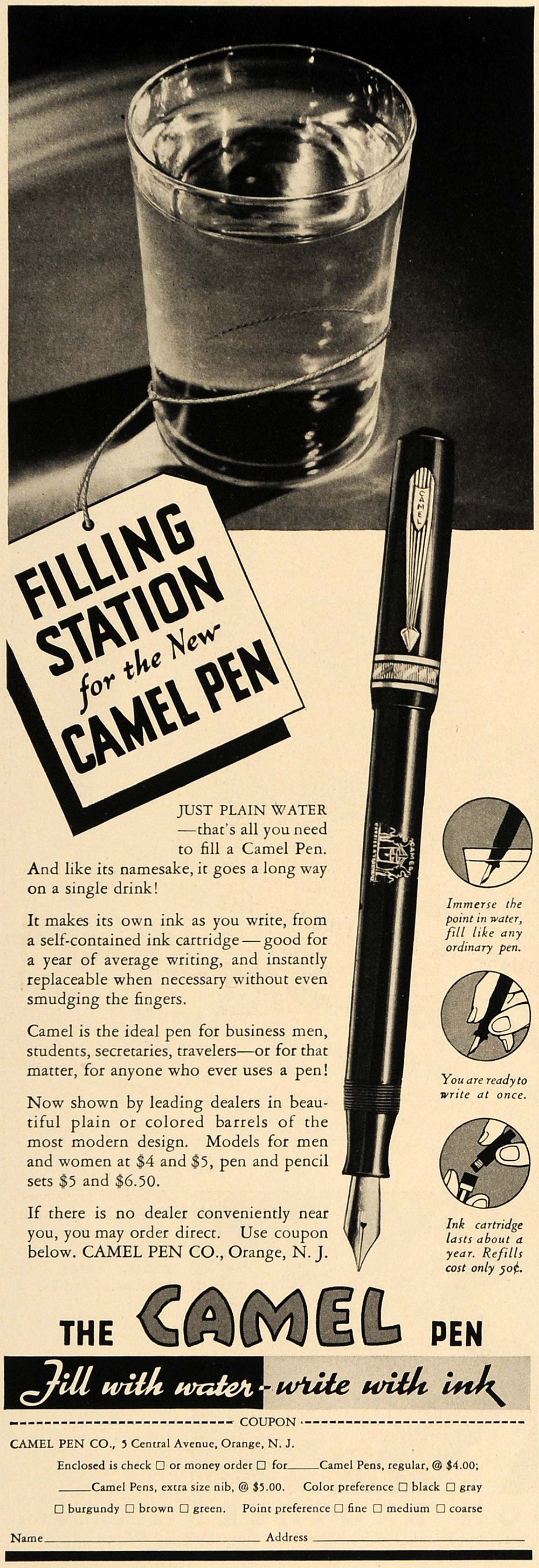This is a black-and-white advertisement for the Camel Pen, presented with an old-fashioned aesthetic, possibly from a tan-colored newspaper. The top section of the advertisement showcases a clear glass of water with an illustrated tag wrapped around it that reads, "Filling Station for the New Camel Pen." Adjacent to the glass, there is a detailed black-and-white drawing of the pen, characterized by its black body and silvery trims around the pen cover. The pen’s unique selling point is described in the image: "Fill with Water, Write with Ink." The central visual theme includes three illustrations demonstrating the pen being dipped in water, then being used to write, and finally, being capped after use. Below these visuals, "The Camel Pen" is highlighted in a playful, cartoonish font, followed by more descriptive text and what appears to be an order form, though the smaller print makes it difficult to read. The advertisement mentions that the company is based out of Orange, New Jersey.